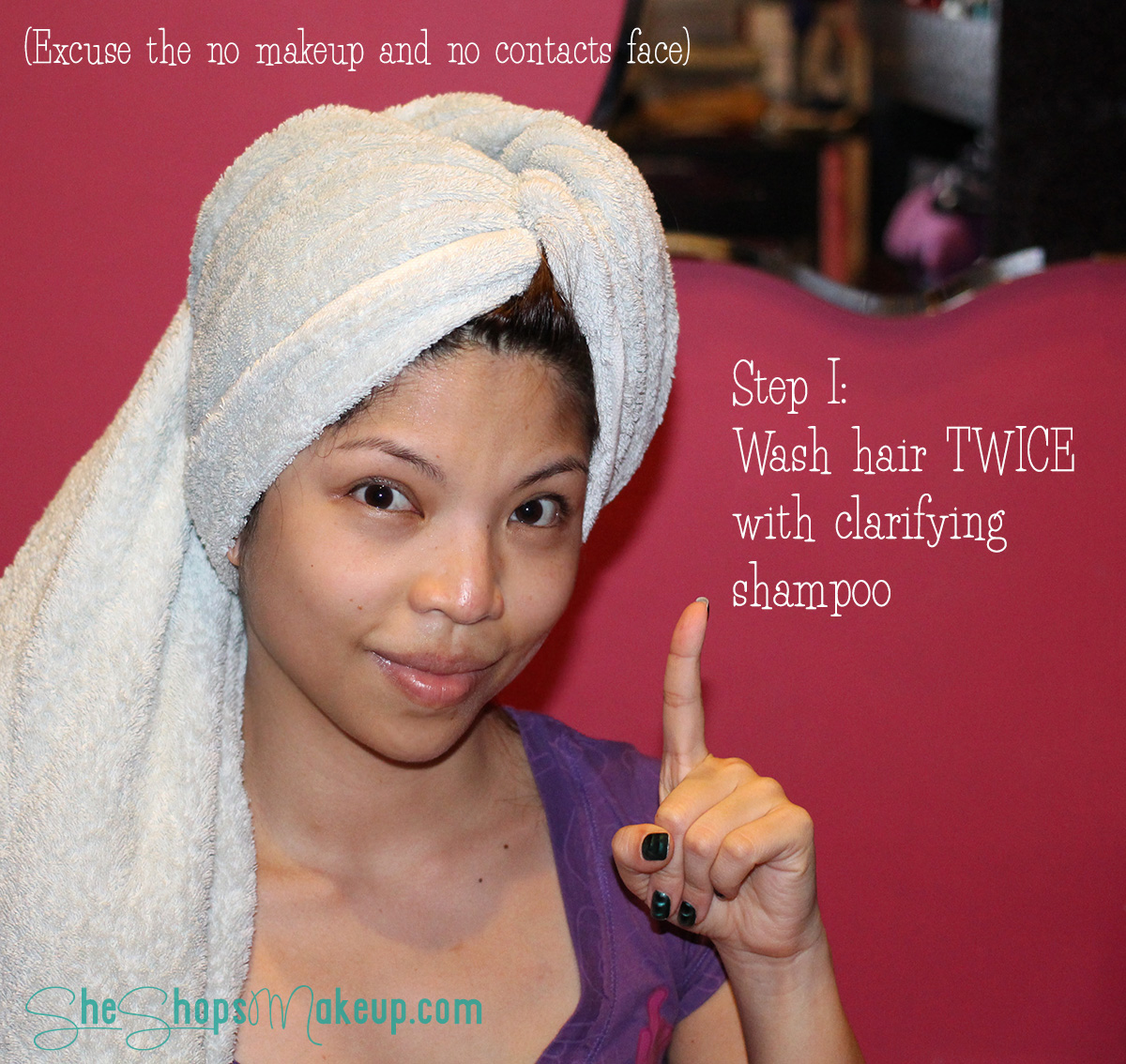The image features an Asian woman with a light complexion, her wet brown hair wrapped in a white towel, indicating she just washed her hair. She is looking into the camera and smiling with her mouth closed, dressed in a purple top. The background is a deep maroon color, and she is standing in what seems to be her bathroom, given the presence of a custom-shaped mirror. In the upper left corner, there is white sans serif text in parentheses that says, "excuse the no makeup and no contacts face." Below this, to the right, another larger, stylized text reads, "STEP ONE: WASH HAIR TWICE WITH CLARIFYING SHAMPOO," which the woman points to with her left index finger while the rest of her hand forms a fist, showcasing her black nail polish. In the bottom left corner, there is green text that reads, "she shops makeup dot com," though this appears to be poorly edited. The overall impression is that of a DIY or amateur tutorial likely intended for social media, emphasizing the first step of a hair care routine.